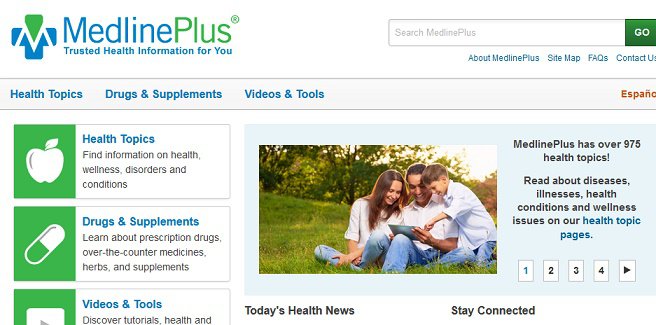The image displays the MedlinePlus website page against a white background. 

In the top left corner, the logo "MEDLINE PLUS" is featured, with "MEDLINE" in blue and "PLUS" in green. Adjacent to the logo, a cross icon is depicted in green and blue. Beneath the logo, the tagline "Trusted Health Information for You" is written in blue.

To the right of the logo, there is a search bar with the placeholder text "Search MEDLINE PLUS" and a green "Go" button. 

Below this search section, several navigational tabs are visible, including "About MEDLINE PLUS," "Sitemap," "FAQs," and "Contact Us."

On the left side below the tagline, additional tabs in blue text read "Health Topics," "Drugs & Supplements," and "Videos & Tools."

Further down, there is a site menu section labelled "Health Topics," featuring a green background with an image of a white apple. The accompanying text reads "Find information on health, wellness, disorders, and conditions." Next, there is a "Drugs & Supplements" section illustrated with a green and white pill on a green background, and the text states "Learn about prescription drugs, over-the-counter medicine, herbs, and supplements." The "Videos & Tools" section is mentioned, but not shown.

On the right side of the image, a family is displayed comprising one female and two boys. Accompanying this image, descriptive text announces, "MEDLINE PLUS has over 975 health topics with information about diseases, illnesses, wellness, conditions, and more on our Health Topics pages." Below this text, pagination numbers from 1 to 4 are seen.

In the bottom left corner, there is a section titled "Today's Health News," while the bottom right corner features a section labeled "Stay Connected."